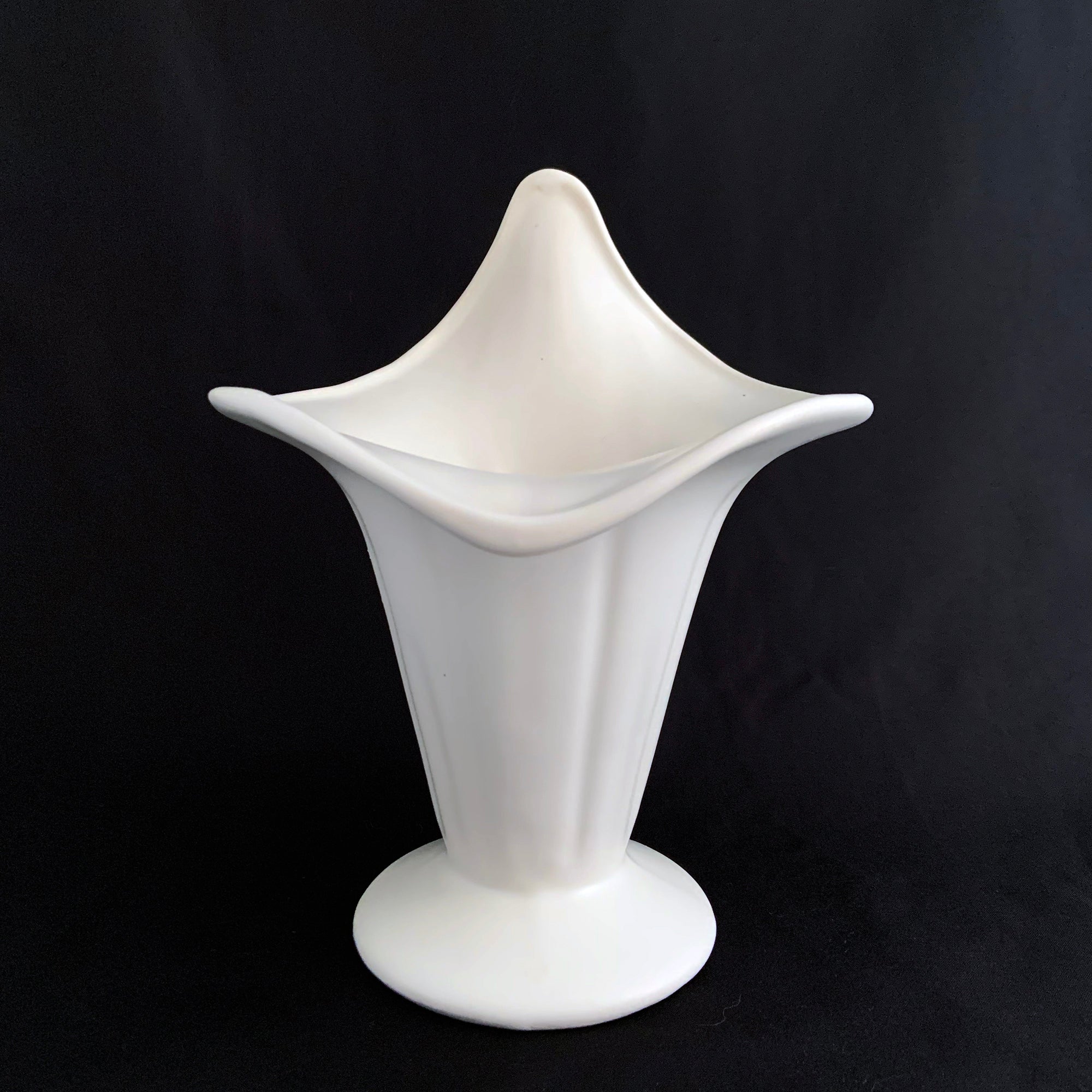This high-quality, professional photograph captures a modern white ceramic vase set against a solid jet black background. The vase, centrally positioned in the square-oriented image, features a rounded, slightly oval base extending horizontally. Crafted from reflective material, the vase's surface appears glazed and slightly shiny. The structure of the vase narrows into a subtle conical shape as it ascends from the base, before flaring outward into an uneven, flower-like opening at the top.

The top of the vase is composed of four major petal-shaped elements with curved tips, resembling the petals of a flower. The rear petal rises higher than the others, creating a dynamic, wavy diamond shape with the front petal dipping lower and the sides transitioning smoothly in-between. The vertical sides of the vase are subtly indented, contributing to its organic, yet contemporary appearance. Its interior, visible only partially from the side angle, displays a reflective surface that contrasts with the outer matte finish. The vase's balanced blend of smoothness and textured indentations adds an artistic touch to this elegant, minimalist piece.